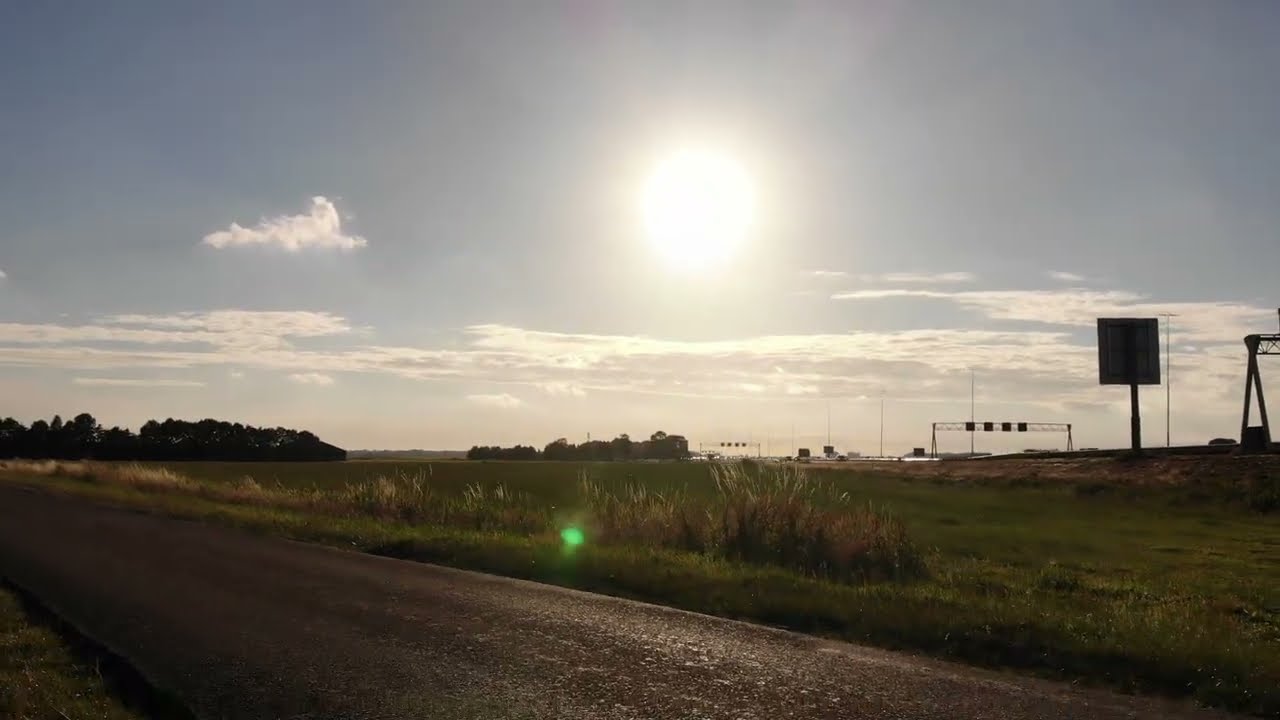The photograph depicts a roadside scene in a natural outdoor setting. In the lower left corner, we can see a small, unmarked, gray-paved road stretching horizontally from the right-hand side to the left-hand side of the image. Adjacent to this road on the right, a vast grassy field spans almost the entire width of the photograph. Most of the grass is green, interspersed with patches of brown, tan-colored hay-like grass.

Further to the right of this grassy expanse, another road structure is partially visible atop a slight elevation, distinguished by its light tan-colored dirt sides. This second road features a metal framework that appears to hold signage or possibly lighting fixtures.

In the background, the landscape features clusters of trees with lush green foliage. The sky above is a clear blue adorned with flat white clouds, and the bright, shining sun is positioned at the center top of the image, casting a natural glow over the entire scene.